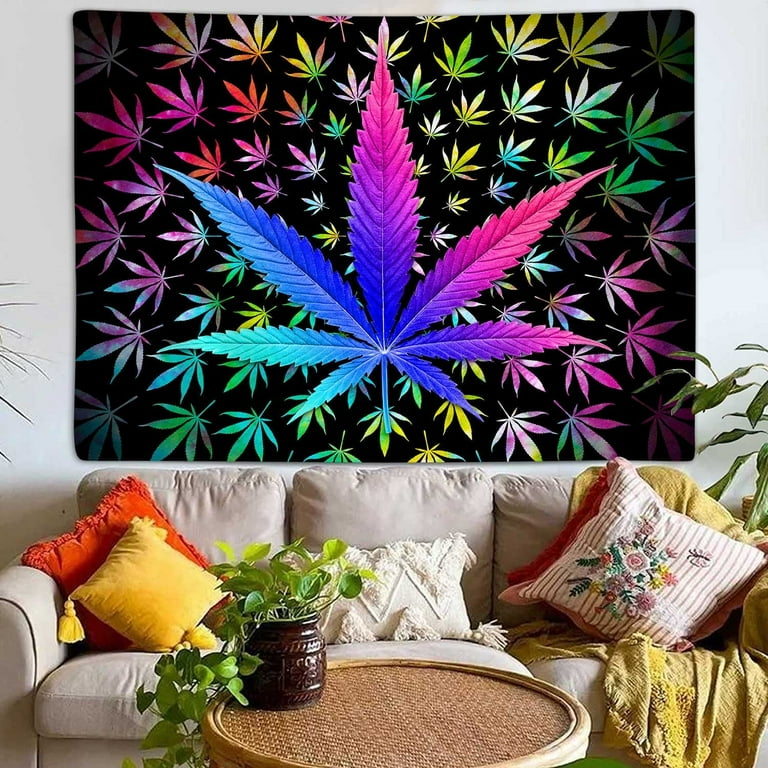This photograph captures a detailed and vibrant close-up view of a living room, focusing mainly on a plush white couch positioned against a light-colored wall. The couch is adorned with an array of colorful throw pillows: a large orange pillow and a smaller yellow pillow with tassels on the left side; a white rectangular pillow with frayed tassels in the middle; and a crocheted white pillow with floral patterns on the right side, which is partially covered by a draped mustard-yellow blanket. 

Above the couch, a large, eye-catching tapestry dominates the scene. The tapestry features a central, multi-colored marijuana leaf with hues ranging from turquoise and deep navy blue to purples and pinks. This leaf is encircled by smaller cannabis leaves radiating outward in a spoke-like pattern. These smaller leaves are depicted in a variety of colors, including yellow, green, pink, blue, and purple, all set against a solid black background, giving the entire piece a psychedelic, cosmic feel.

In front of the couch sits a round wicker coffee table, on which rests a brown ceramic planter housing lush green ivy, adding a natural touch to the vibrant interior. The combination of the colorful tapestry, the eclectic mix of plush pillows, and the green plant creates a rich, textured, and lively atmosphere in this cozy living room setup.